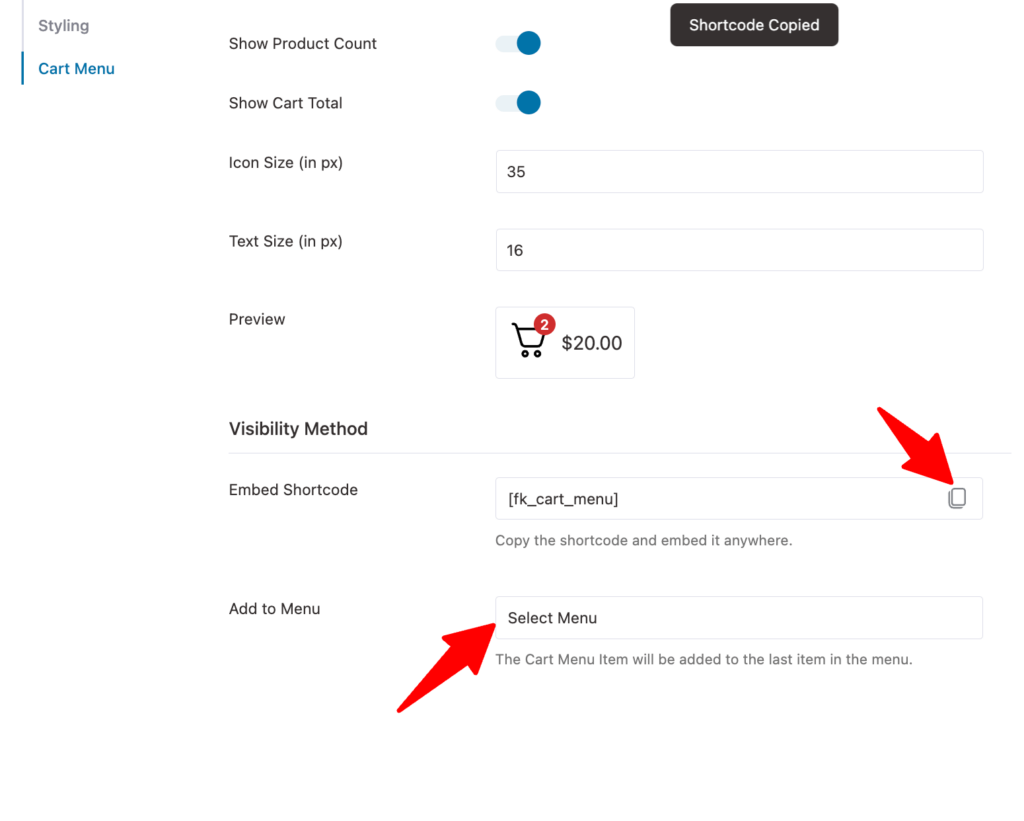The image depicts a computer screen displaying a user interface for customizing a shopping cart widget. 

At the very top left, there's a blue-highlighted "Cart Menu" tab, indicating the current selection. Below this, a black label states "Shortcode Copied." To the right, toggle switches are present for enabling "Show Product Count" and "Show Cart Total." These are accompanied by input fields for setting "Icon Size (in pixels)" and "Text Size (in pixels)," with values entered as 35 and 16, respectively.

Further down, there's a section labeled "Preview," which showcases an image of a shopping cart icon. The cart contains a red circle with the number "2" and a total price displayed as "$20." 

Below the preview, a segment titled "Visibility Method" offers options for displaying the cart, highlighting the "Embedded Shortcode" method. An example shortcode is provided within a white rectangular input box. Next to this, instructions read "Copy the shortcode and embed it anywhere."

Additionally, an "Add to Menu" option is available, suggesting users can select a menu to place the cart. Red arrows in the image point towards the respective "Copy" button and the "Select a Menu" dropdown, as well as towards the cart menu tab, indicating steps to follow for customization.